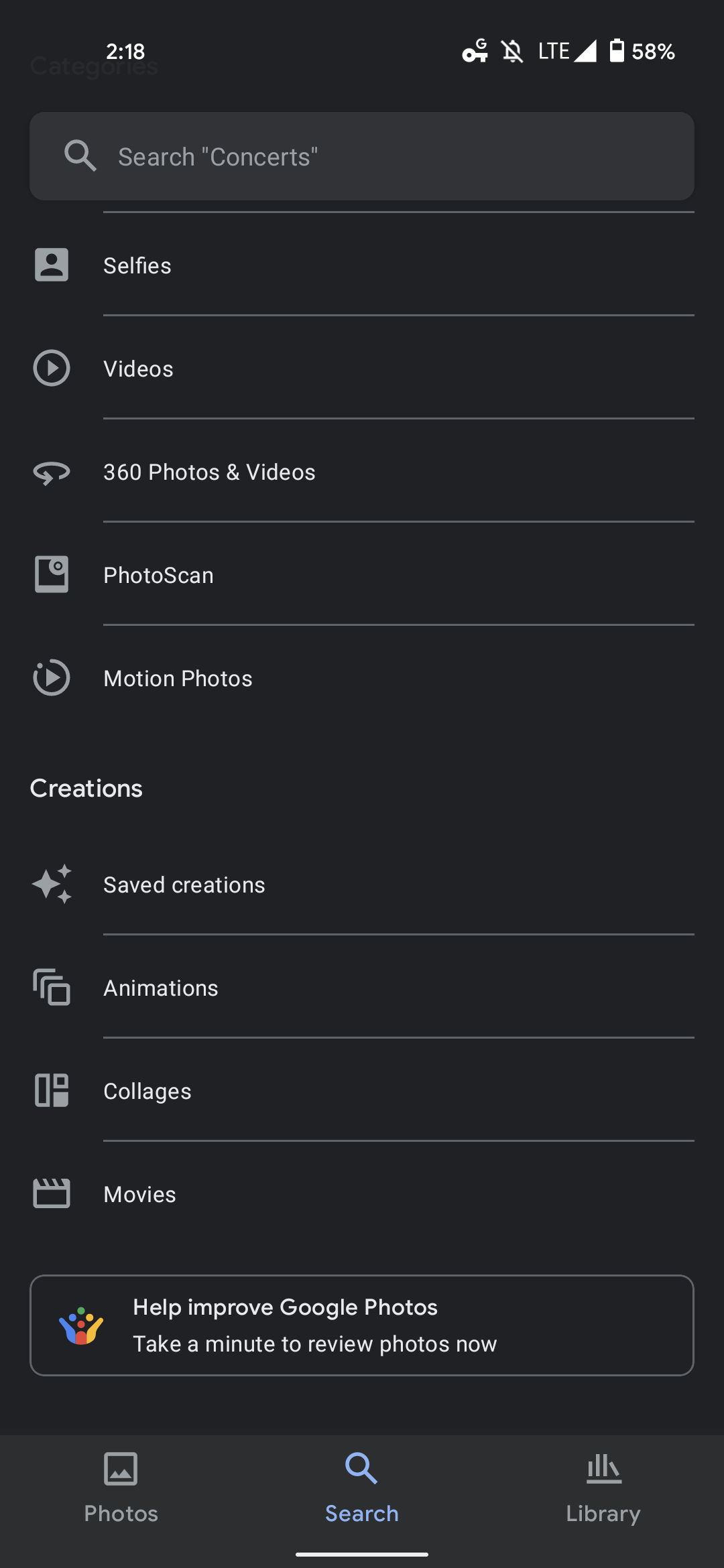The image depicts a smartphone screen displaying the Google Photos application with a predominantly black background. In the upper left corner, the number "218" is visible, while the upper right shows a battery icon indicating 58% charge, beside an LTE signal icon, a muted bell symbol, and a "G" sign.

Beneath this, a dark gray banner houses a gray search icon next to the text "Search Concerts." The main content area starts with the header "Selfies" in white text, accompanied by a gray icon representing a person. Following this, the section titled "Videos" features a gray circle with a gray triangle icon.

Next is the "360 Photos and Videos" category, symbolized by a gray 3-quarter circle with an arrow, followed by "Photo Scan," represented by a gray square with a circle and a dot in the center. The "Motion Photos" section displays a gray 3-quarter circle with a gray triangle.

Under a fine gray divider line is the "Creations" section, starting with "Saved Creations," illustrated by three small stars. The "Animations" category is next, shown with three overlapping boxes. Another fine gray line leads to "Collages," depicted with a long rectangle, a small square outline, and a solid gray square.

Below another fine divider, the "Movies" category is marked with a gray square with a black center and diagonal lines at the top. A banner outlined in gray reads "Help Improve Google Photos. Take a minute to review photos now," showcasing the Google color dots and a small icon in blue, red, and gold.

At the bottom of the screen, the navigation bar displays "Photos" in gray with a corresponding square icon on the left, "Search" in blue with a blue search bar in the middle, and "Library" on the right, indicated by a gray horizontal line with small books.